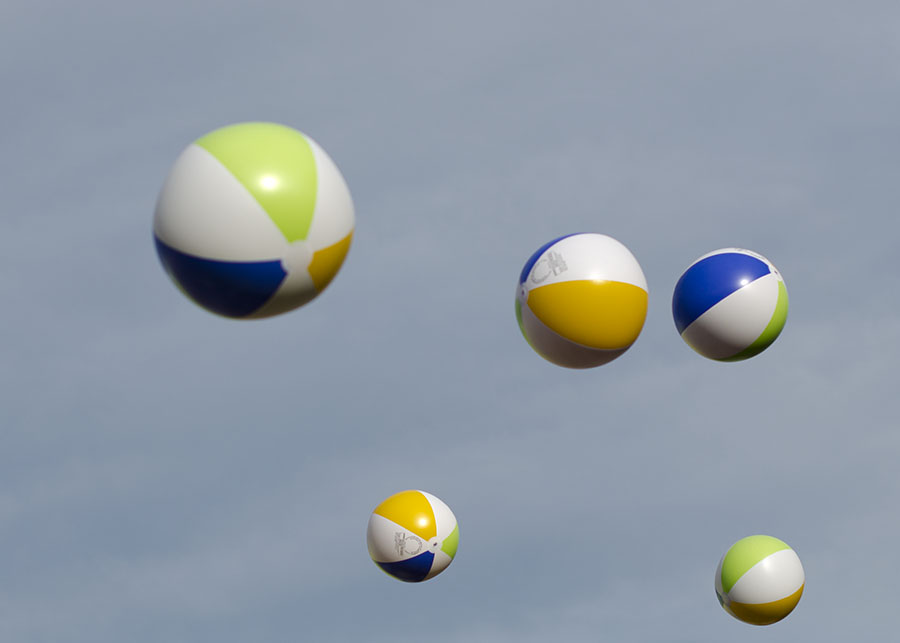The image depicts five beach balls of varying sizes in flight against a grayish blue sky, which may not be real but rather an artificial backdrop. Each beach ball features the same coloration: white segments alternating with green, navy blue, and orange-yellow stripes. A small, unreadable logo is present between some of the colored sections on each ball. The balls are positioned at different heights and distances; one prominent ball is near the top right corner, with another larger one slightly lower and to the center. Two are situated side-by-side in the top right region, with a smaller ball appearing blurry and closer on the left. Additional balls are spread out across the middle to bottom area of the composition, adding to the dynamic sense of movement. Reflective light spots on different segments suggest sunlight from an out-of-frame source, enhancing the visual depth of the image. Overall, the scene has a somewhat surreal quality, potentially pointing to a digitally generated composition.